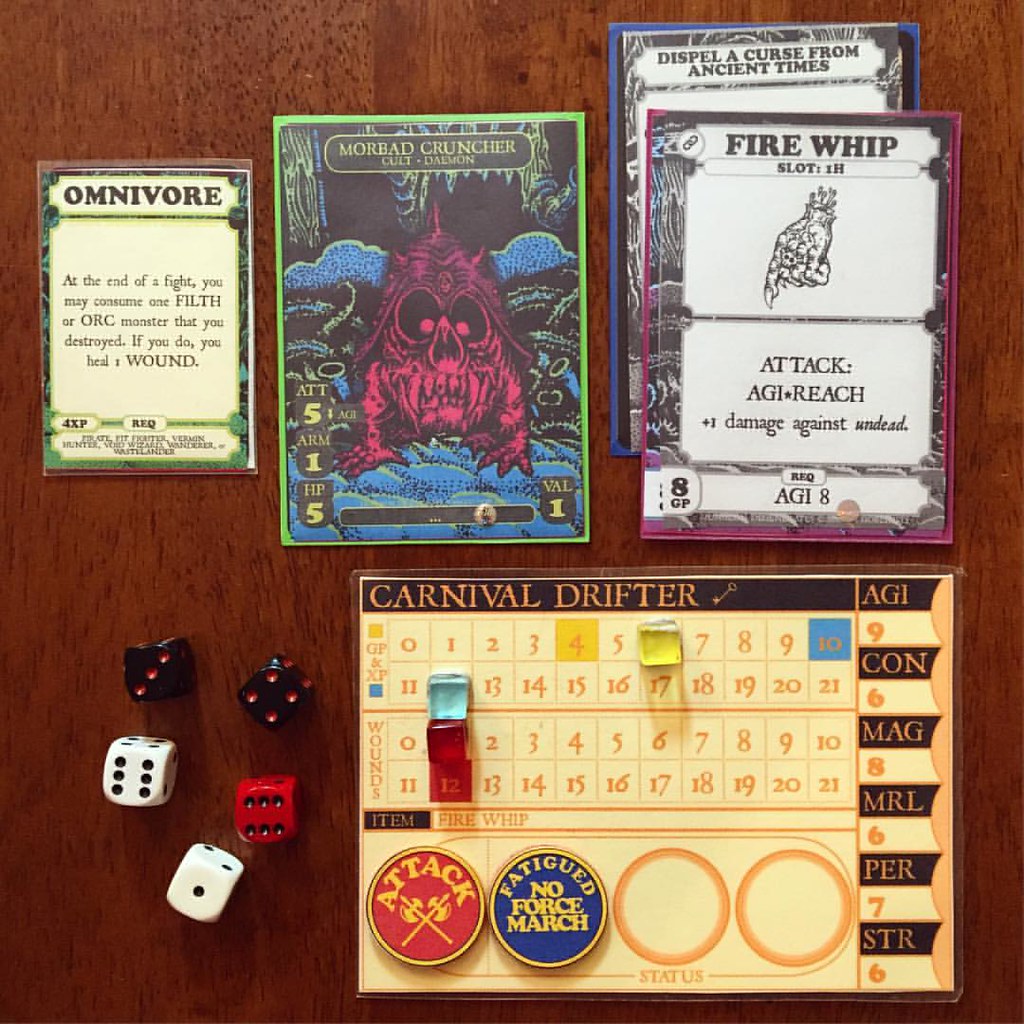The image depicts an intricately setup for a board or role-playing game laid out on a brown wooden table. The focal point is a character sheet titled "Carnival Drifter" on a yellow board with a black bar at the top and the title in gold lettering. This sheet features numerical tracks running horizontally from 1 to 20, with yellow, light blue, and red square markers placed on numbers 6, 12, and 1, respectively. Below these, there are various stat sections denoted by labels such as AGI, CON, MAG, MRL, PER, and STR, alongside bead counters to track scores. On the left of the markers, five six-sided dice are present: two black dice showing 3 and 4, two white dice showing 6 and 1, and a single red die showing 6.

In the upper left corner of the setup, there's a rectangular card labeled "Omnivore" bordered in green, detailing a special ability to heal by consuming a defeated filth or orc monster. To the right, a larger card titles "Morbad Cruncher" portrays a red demon with blue wings and game statistics, possibly indicating either an enemy or player character. Adjacent to this is another card named "Fire Whip," highlighting an attack move with instructions and effects on undead entities. A third card, "Dispel a Curse from Ancient Times," completes the set of cards on the top right.

Overall, the image conveys a detailed and engaging gaming setup with various cards, dice, markers, and a wooden background, showcasing a complex and intriguing game mechanics.